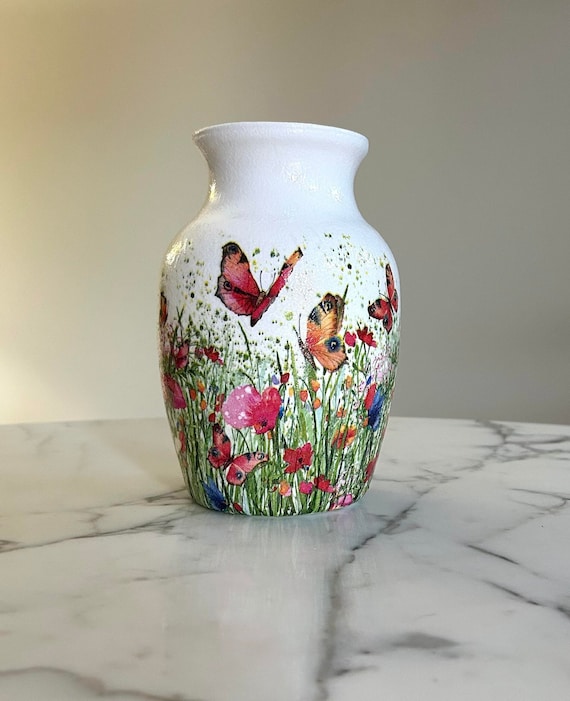The photograph captures an intricately painted white vase, likely made of clay, set against an indoor display with a white wall in the background. The vase stands on a round marble tabletop characterized by its grey and black veins. The vase itself is adorned with a vibrant and detailed floral and natural scene. Among the painted decorations, there are numerous individual blades of green grass, various flowers, and several butterflies. Flowers in hues of pink, orange, yellow, blue, and red cascade around the vase, contributing to its picturesque appearance. Butterflies with pink, orange, yellow, and black wings are depicted both flying and resting on the flowers and grass, adding a lively touch to the artistic display. The overall composition and the ceramic's fine details suggest it could be a decorative item or something available for sale.